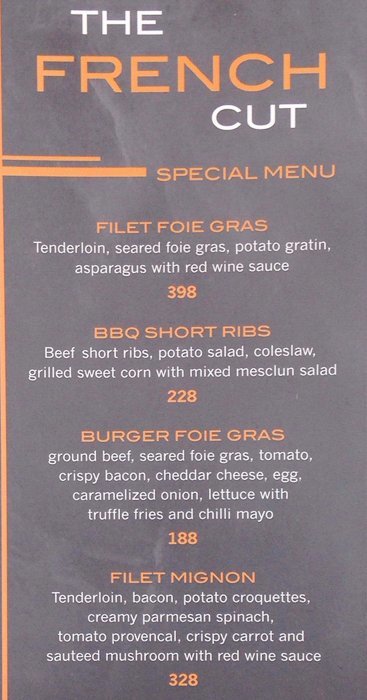This image features a visually striking menu page from a restaurant called "The French Cut." The menu has a sophisticated gray background accentuated by vertical and horizontal lines in various shades of orange. The title at the top reads "The French Cut," with "French" highlighted in orange, while the rest is in white. Below this, a horizontal line extends halfway across the page, beneath which the words "Special Menu" are prominently displayed. 

The menu lists the following items, each detailed with ingredients and pricing:

1. **Filet foie gras**
   - **Description:** Tenderloin seared foie gras, potato gratin, asparagus with red wine sauce
   - **Price:** $3.98 in red letters

2. **Barbecue short ribs**
   - **Description:** Beef short ribs, potato salad, coleslaw, grilled sweet corn with mixed mesclun salad
   - **Price:** $2.28 in orange letters

3. **Burger foie gras**
   - **Description:** Ground beef, seared foie gras, tomato, crispy bacon, cheddar cheese, egg, caramelized onion, lettuce with truffle fries and chili mayo
   - **Price:** $188 in orange letters

4. **Filet mignon**
   - **Description:** Tenderloin, bacon potato croquettes, creamy Parmesan spinach, tomato Provencal, crispy carrot, and sautéed mushrooms with red wine sauce
   - **Price:** $3.28 in orange letters

The use of color to differentiate text and prices adds a sophisticated and visually appealing touch to the menu, enhancing its overall elegance and readability.